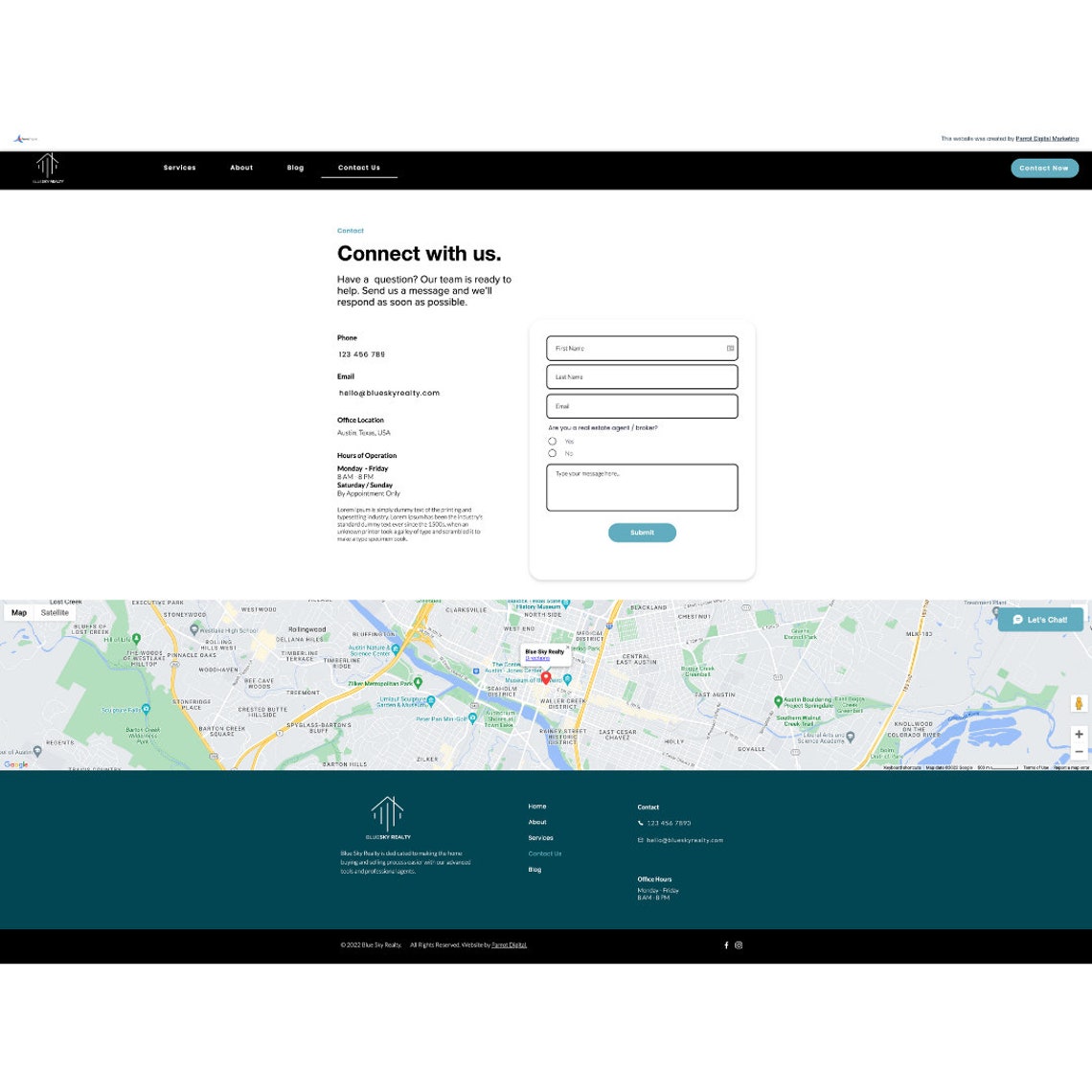Screenshot of a website showcasing its "Contact Us" form. The upper section features a sleek black navigation bar, adorned with a small logo in the left corner, followed by menus for "Services," "About," "Blog," and a highlighted "Contact Us" tab. Dominating the page is a comprehensive contact form, allowing users to reach out to the website's owners. The contact section provides additional details, including the company's phone number, email address, office location, and hours of operation. Beneath the form, a rectangular map snippet visually pinpoints the business location. The bottom section of the page displays another navigation bar set against a dark green background, featuring the company logo once more alongside a detailed list of website sections and more contact information.